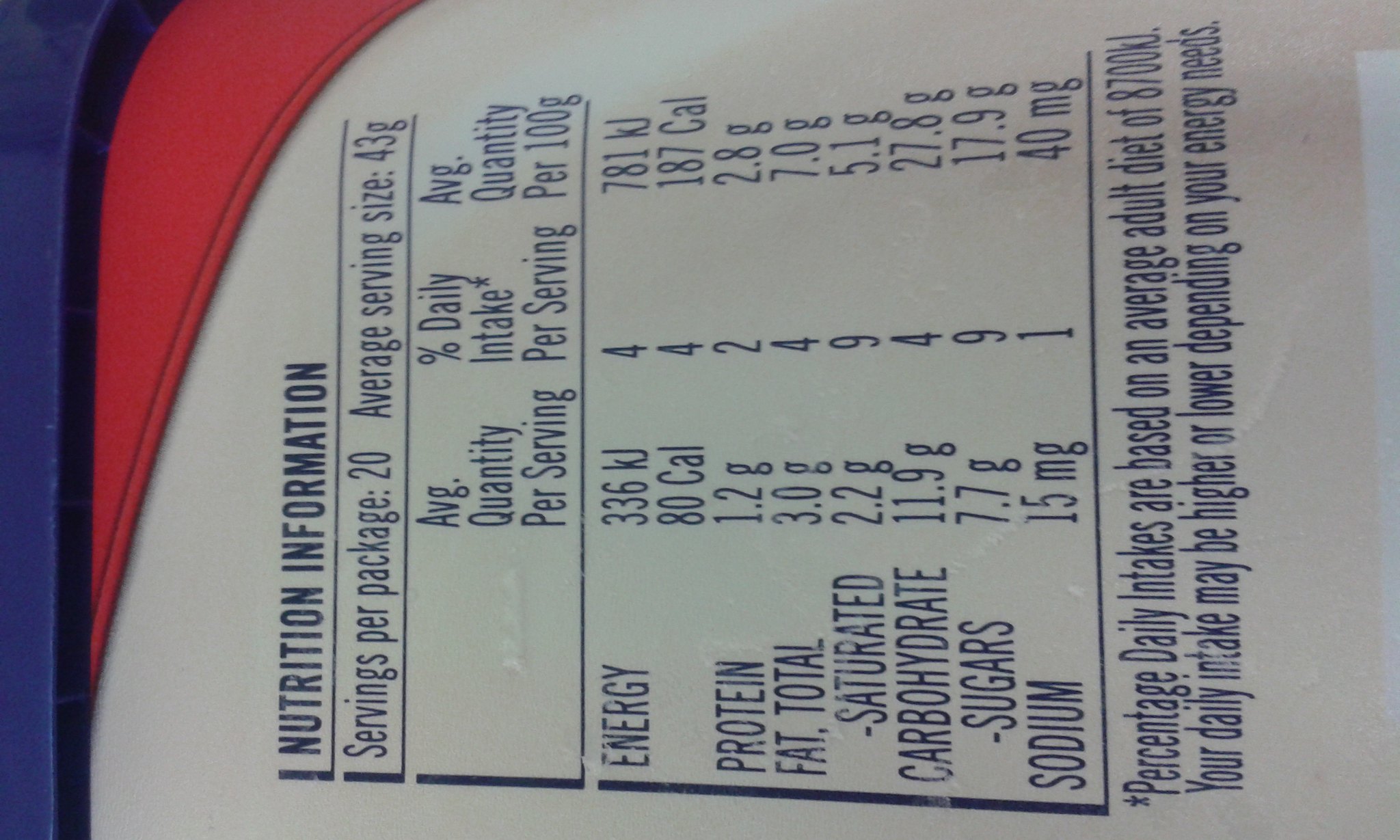This image is an up-close photograph of a nutrition information label, which has been rotated 90 degrees anti-clockwise, requiring viewers to tilt their heads to the left to read it properly. The label is predominantly white with dark blue writing, featuring a red swoop on the left side, likely indicating part of the packaging design. At the top of the label, the heading reads "Nutrition Information," which is underlined. Below this, the label lists "Servings per package: 20" and "Average serving size: 43 grams."

The nutritional values are divided into three columns: the first column details the "Average Quantity per serving," listing the following nutrients: Energy (336 kilojoules or 80 calories), Protein (1.2 grams), Fat - Total (3 grams), Saturated Fat (2.2 grams), Carbohydrates (11.9 grams), Sugars (7.7 grams), and Sodium (15 milligrams). The second column, labeled "Percentage Daily Intake per serving," provides the respective percentage values: 4% for Energy, Protein, Total Fat, and Saturated Fat; 9% for Carbohydrates and Sugars; and 1% for Sodium. The third column shows the "Average Quantity per 100 grams," which includes the quantities: Energy (781 kilojoules or 187 calories), Protein (2.8 grams), Fat - Total (7 grams), Saturated Fat (5.1 grams), Carbohydrates (27.8 grams), Sugars (17.9 grams), and Sodium (40 milligrams).

Beneath these columns, there is a note marked with an asterisk, stating, "Percentage daily intakes are based on an average adult diet of 8,700 kilojoules. Your daily intake may be higher or lower depending on your energy needs." There are no indications of the USDA label or additional details about the food product itself.